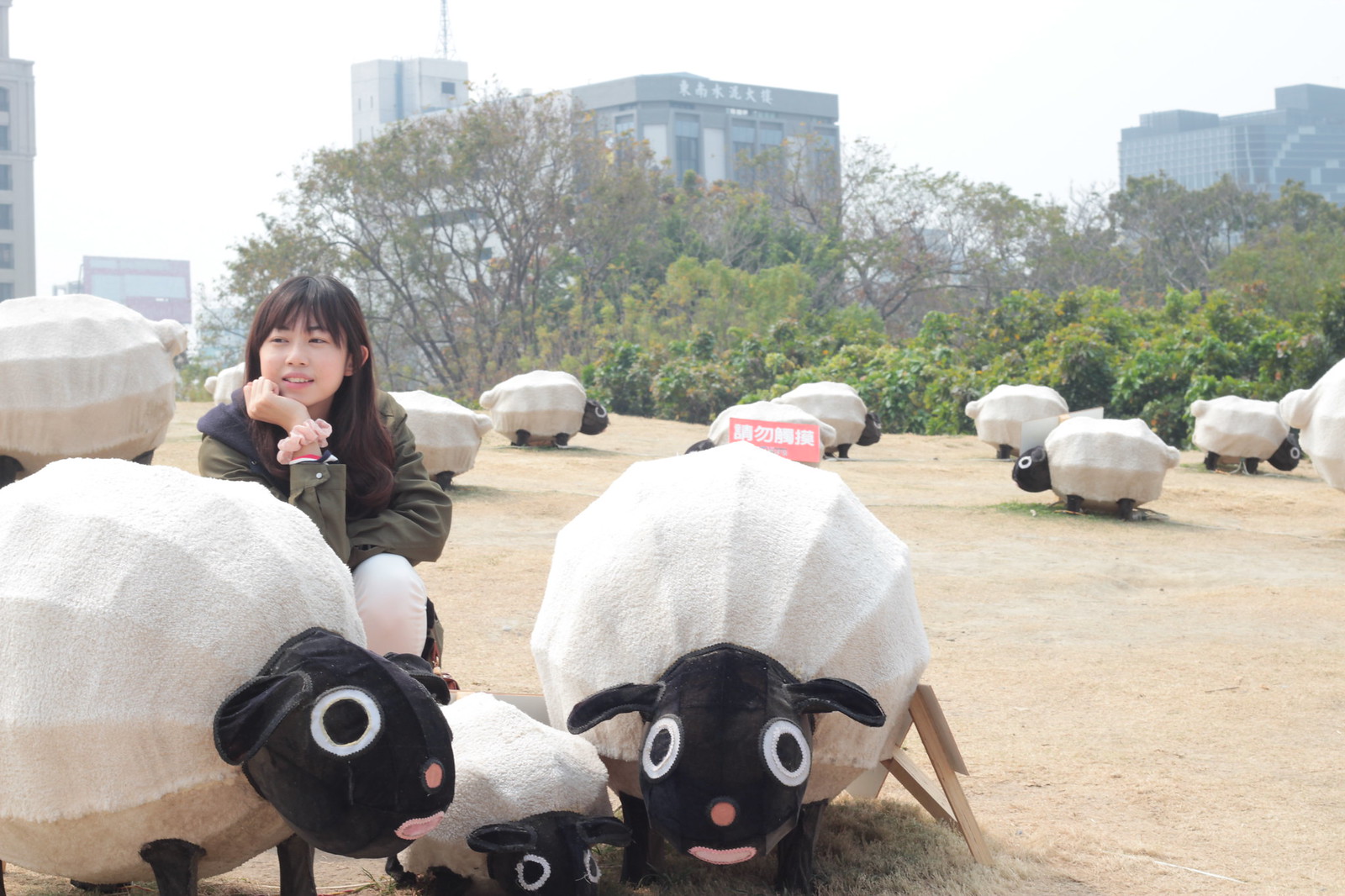The image depicts a potentially Asian outdoor art installation featuring numerous crafted sheep sculptures scattered across a brown, sandy field. These sheep figurines are designed with white bodies, black heads, and floppy ears, along with distinctive pink noses and mouths. Their legs appear to be made from natural light wood. In the background, several skyscrapers are visible against a white sky, partially obscured by green trees. A young girl, likely aged between 15 to 20, of East Asian descent, with black hair and dressed in a dark green jacket with black trim, and white pants, is kneeling beside one of the sculptures. She has her right hand under her chin and a scrunchie around her right wrist, gazing thoughtfully into the distance. The photograph captures a juxtaposition of urban and artistic elements within a serene, open space.